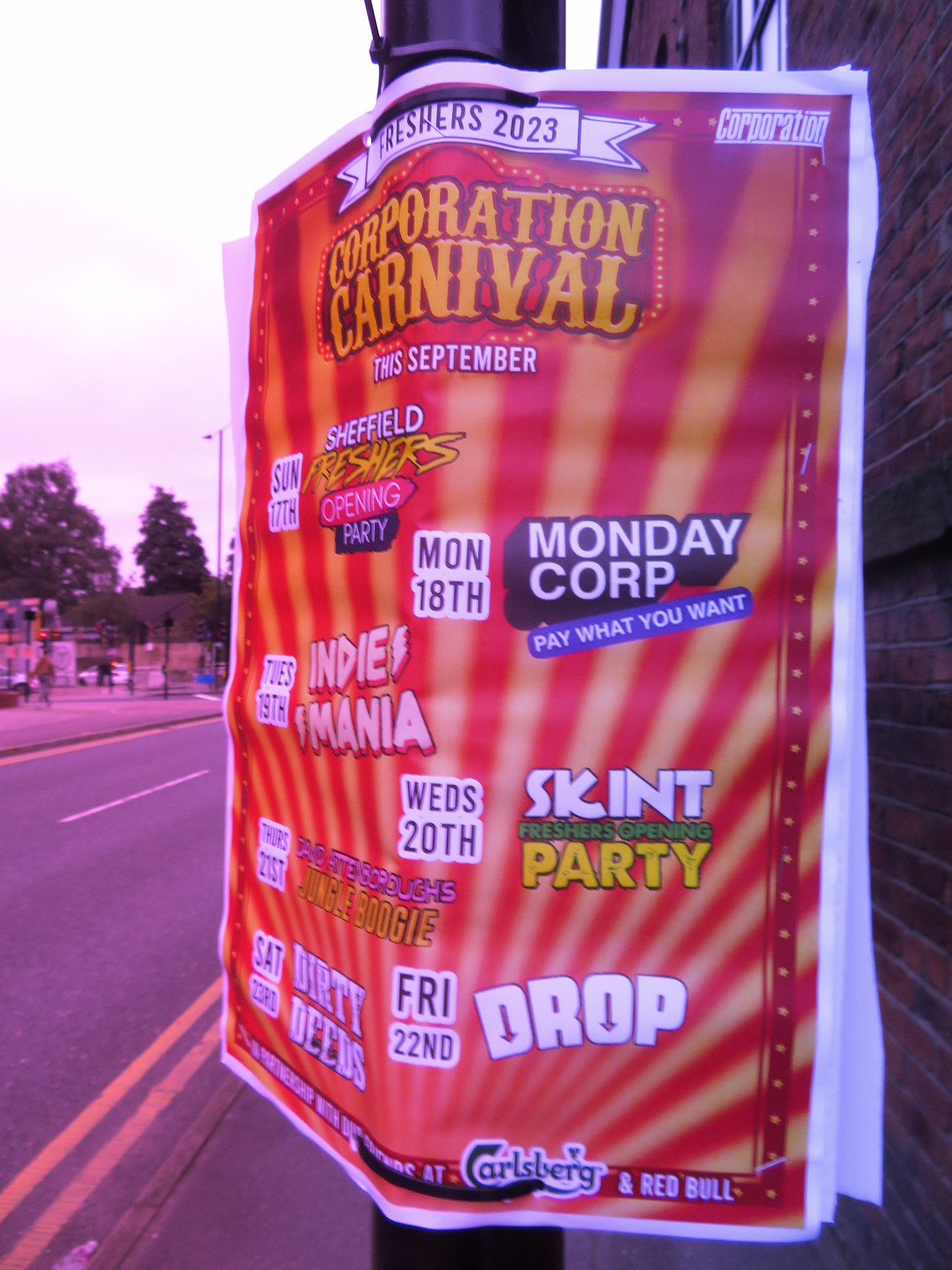The image is a portrait-mode photograph of a flyer that is taped or zip-tied to a street pole. The main focus is the vibrant flyer, which has a red background with bold yellow text at the top reading "Corporation Carnival." Beneath it, in white text, is "This September," followed by a list of event dates and descriptions. The flyer schedules a series of events starting Sunday the 17th with the "Sheffield Freshers Opening Party," continuing with "Monday Corp. Pay What You Want" on the 18th, "Indie Mania" on the 19th, "Skint Freshers Opening Party" on the 20th, "Bad Attenborough's Jungle Boogie" on the 21st, "Drop" on the 22nd, and concluding with "Dirty Deeds" on Saturday the 23rd. At the very top, a banner states "Freshers 2023." The poster also features logos of sponsors, including Carlsberg and Red Bull, in the bottom right corner.

In the background to the right, there is a brick building with a window. To the left of the pole, the street is visible with yellow and white lines, and further left, a blurry view of another sidewalk, where a person, some cars, foliage, and trees can be seen. The photograph was clearly taken outside with the photographer standing on a sidewalk.